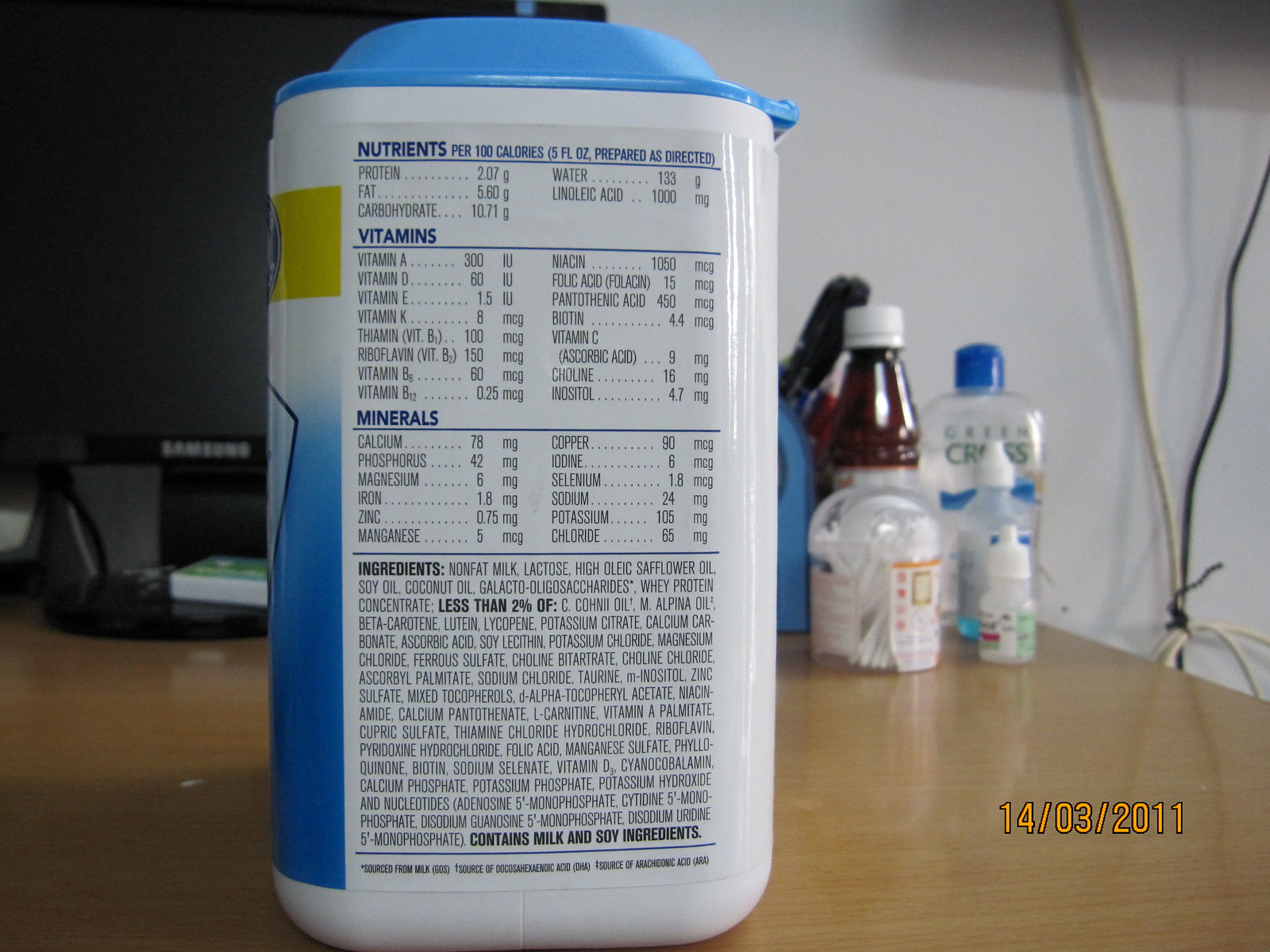This image features a white container with a light blue lid, likely a protein drink mix or nutritional supplement, prominently placed in the foreground. The container's label emphasizes its rich content of various nutrients, vitamins, and minerals. Detailed ingredient information indicates that the product includes healthy components, with water listed as a primary ingredient. The label, colored blue towards the bottom, has a goldish-greenish stripe along the top edge.

The container rests on a wooden counter, surrounded by assorted toiletries including other bottles and a container of Q-tips. In the background, a black device, possibly by Samsung, is partially visible. Additionally, there are wires dangling from the wall, neatly tied together. This photograph was taken on March 14, 2011.